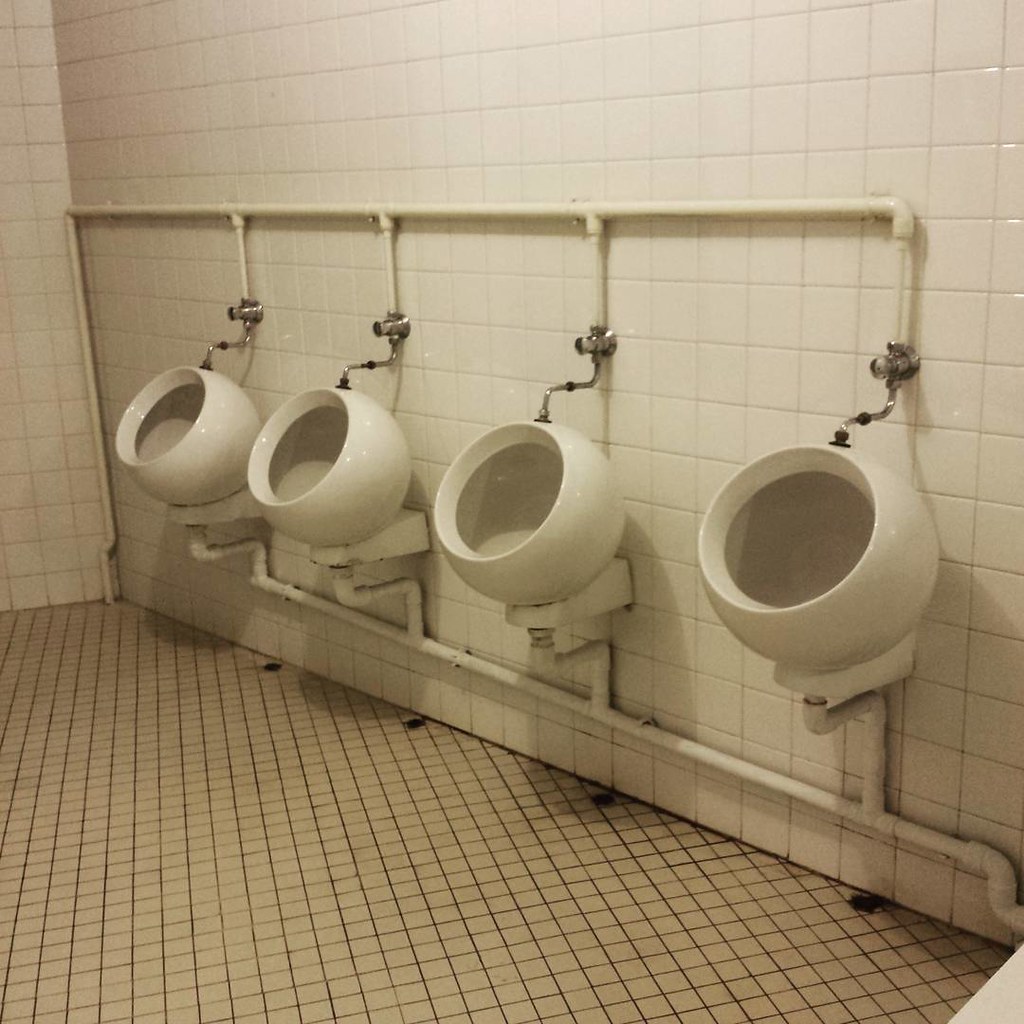The image depicts a dirty public restroom, likely in Japan, featuring four high-mounted urinals aligned against a wall. These urinals, resembling either cement mixers or vintage 1950s hair dryers, have a distinctive round bowl design, which sets them apart from typical urinal shapes. Each urinal connects to a plumbing system through a small silver hose and has a handle for flushing. The restroom's walls are covered in shiny, white, standard square tiles, reminiscent of shower tiles, while the floor consists of smaller beige tiles with dark brown marks and dingy grout, reinforcing the overall unkempt appearance. Despite the cleanliness of the urinals themselves, the floor appears particularly filthy. The space is devoid of any other fixtures or decorations.